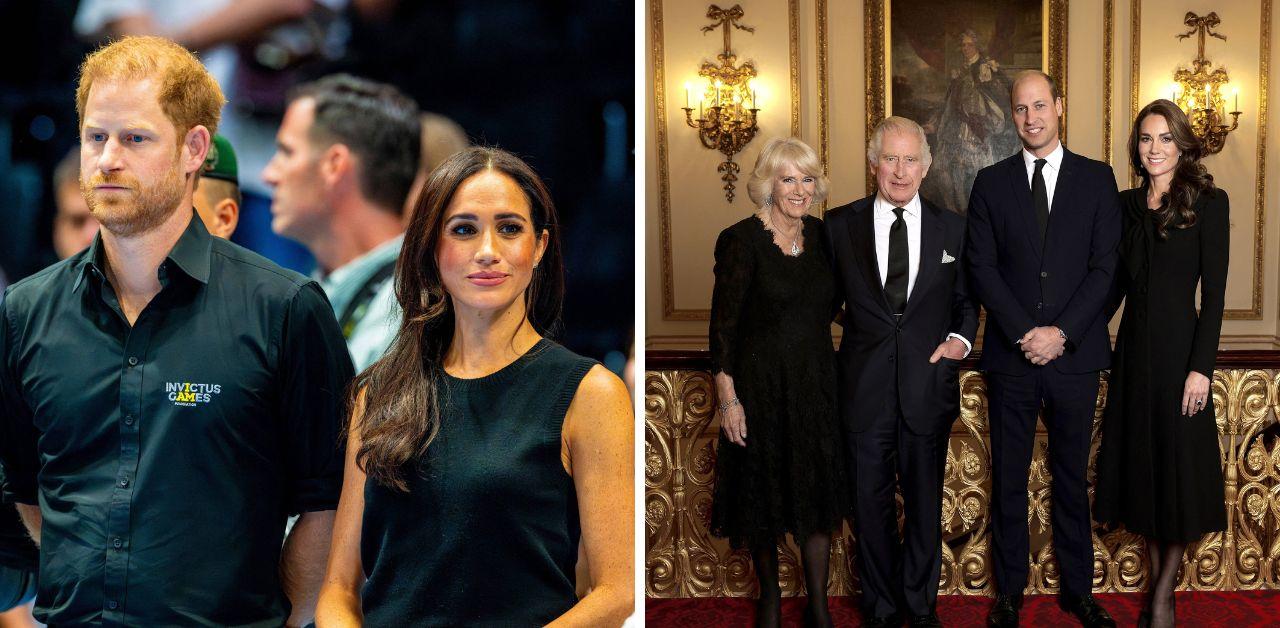The image is a horizontally rectangular, full-color composite made up of two square photographs with a white vertical border between them. In the left photograph, Prince Harry and Meghan Markle are seen from the waist upwards. Prince Harry is wearing a green button-up shirt with the "Invictus Games" logo on the chest, staring straight ahead. Meghan Markle, in a green sleeveless dress, has long brown hair cascading below her shoulders and holds a closed-mouth smile. They seem to be at an event, standing slightly apart and looking in opposite directions.

The right photograph features four members of the royal family, visible from their ankles upwards. From left to right, the figures are: a woman in a black dress who is likely Kate Middleton; Prince William in a black suit with a black tie and white button-up shirt; King Charles, dressed similarly in a dark blue suit; and an elderly woman with short blonde hair, likely Camilla, in a long-sleeved black dress. They stand indoors, adorned in formal attire, against a backdrop decorated with gold and a painting of another king between Charles and William, suggesting a regal setting, possibly a castle.